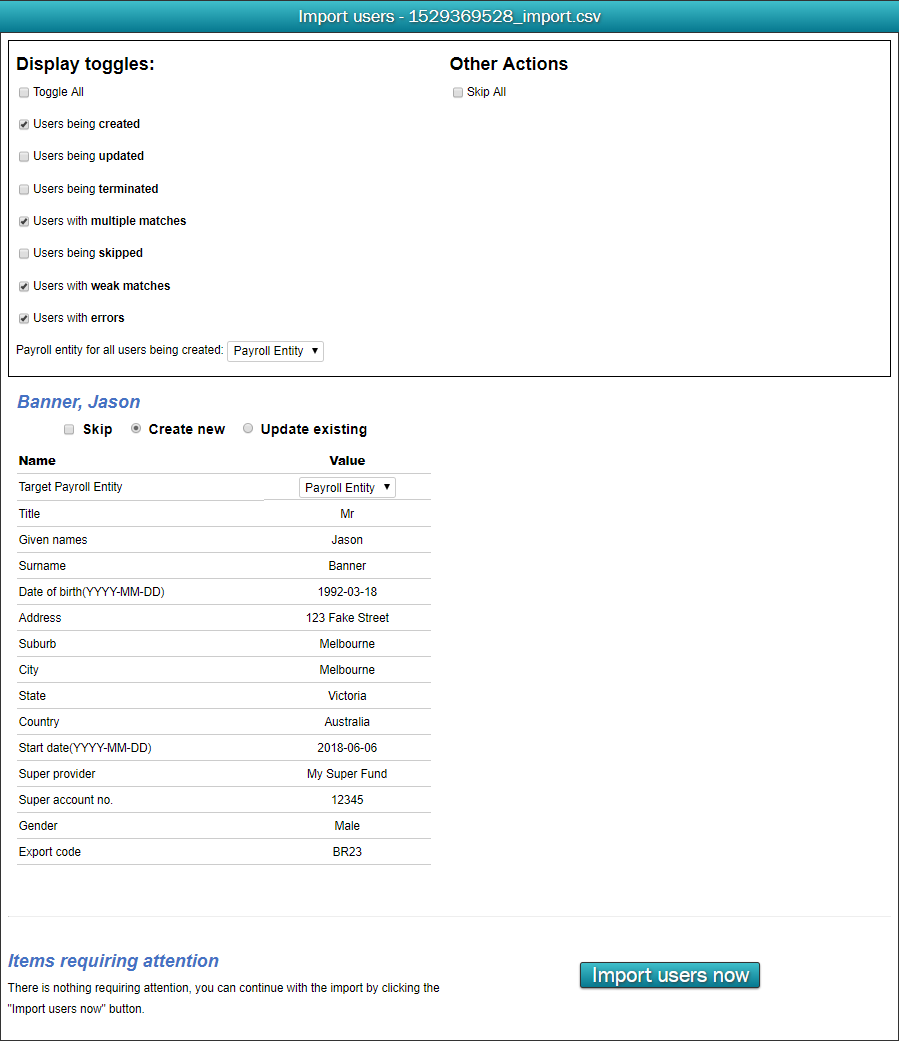The image shows a screenshot of a computer application interface for importing users. At the top of the interface, there is a gray or teal rectangle displaying the label "import_users-1529369528_import.csv". Below this, there is a section labeled "Display Toggles" with an option "Toggle All" which is not checked. Below the display toggles, there are several options with checkboxes on the left and descriptions on the right:

- "Users being created" is checked.
- "Users being updated" is unchecked.
- "Users being terminated" is unchecked.
- "Users with multiple matches" is checked.
- "Users being skipped" is unchecked.
- "Users with weak matches" is checked.
- "Users with errors" is checked.

Further down, there is a label "Payroll entity for all users being created" followed by a field labeled "Payroll Entity". At the top of this section, there is another heading "Other Actions" with an option "Skip All" that is not checked. There is also a mention of "Banner JSON". Towards the bottom, likely indicating the user's name. Finally, at the bottom of the interface, there is a teal rectangle button labeled "Import Users Now".